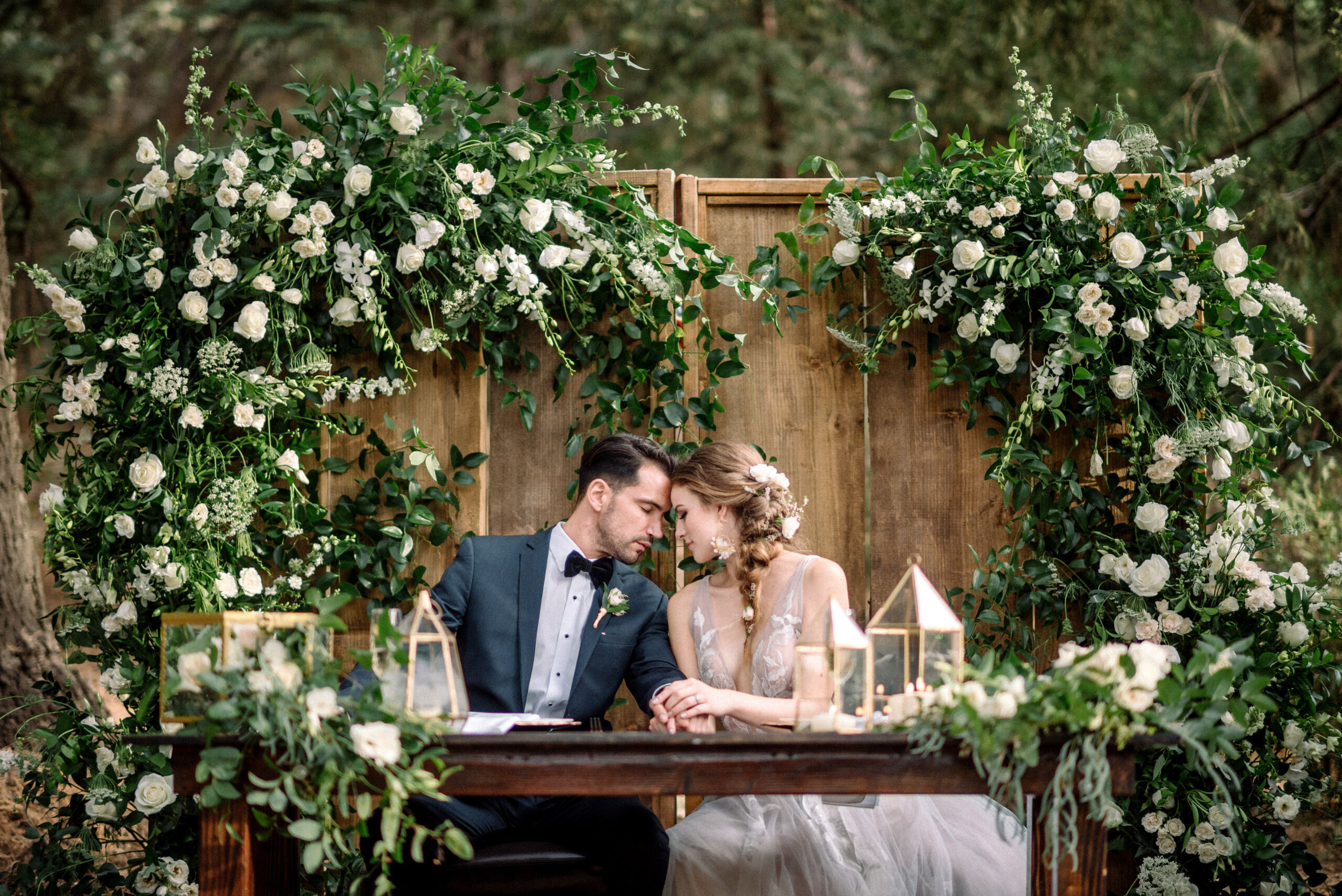The photograph captures an intimate moment between a bride and groom on their wedding day, seated at a wooden table. The groom, donned in a charcoal gray suit with a black bow tie and a flower on his lapel, sits on the left. The bride, in a sheer white lacy gown that shows a touch of cleavage, sits on the right. Her light brown hair is intricately braided and adorned with small white flowers, cascading over one shoulder. Both of them have their foreheads gently touching, eyes closed, savoring the moment, as they clasp hands—his left hand enveloped by both of hers. Behind them, two large wooden panels form a backdrop, lavishly decorated with white roses and lush greenery that extend down the sides in a heart-shaped arrangement. Enhancing the romantic ambiance, the wooden table in the foreground is accented with geometric glass lanterns featuring golden details. The rich, green, foresty background further adds to the serene and enchanting feel of the setting.